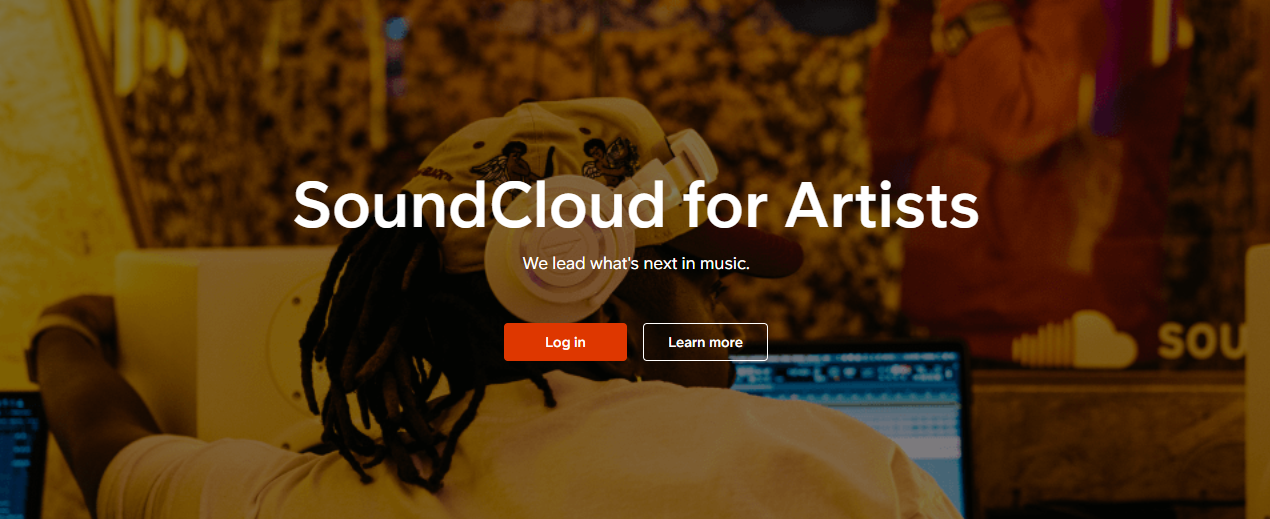The image is a screenshot of the SoundCloud webpage tailored for artists. At the top, the header reads "SoundCloud for Artists," with the words "SoundCloud" and "Artists" each starting with a capital letter ('S' and 'C' in 'SoundCloud' and 'A' in 'Artists'). Directly beneath this, the tagline "We lead what's next in music" is prominently displayed. 

On the right side of the page, there are two distinctive buttons: one in red labeled "Login," and another in black labeled "Learn More." 

The central portion of the image features a photograph of a man sitting, possibly on a sofa or at a table. He is wearing a white T-shirt and white headphones, suggesting he is listening to music. His hair is styled in dreadlocks, and his gaze is directed slightly to the right, likely toward a computer screen.

To the right of this photograph, the SoundCloud logo is visible. The logo, which resembles a half cloud composed of partially filled bars, emphasizes the brand's identity and association with sound and music streaming.